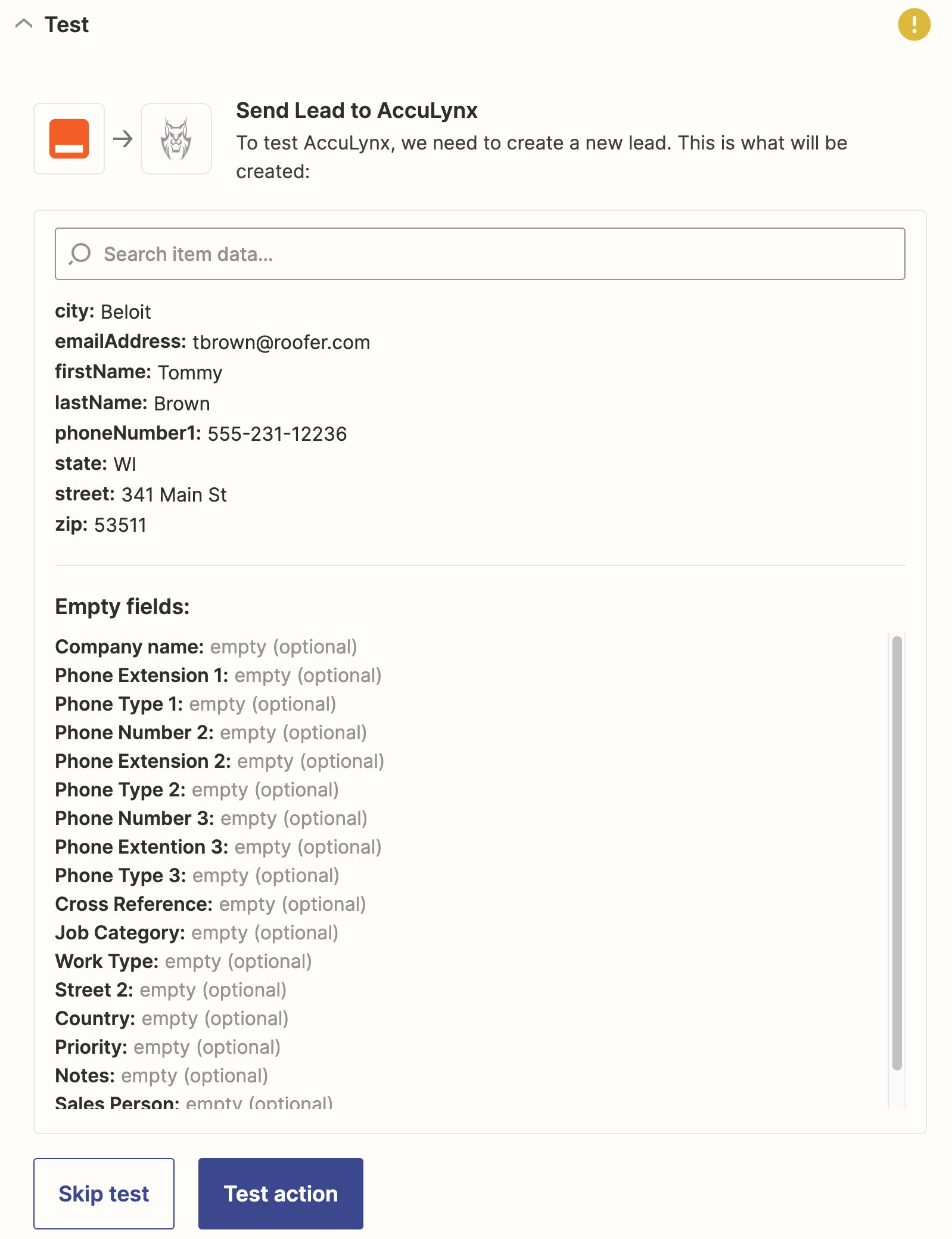Screenshot Caption:

This screenshot appears to be taken from either a computer or phone screen of an interface, displaying a form or setup screen for "AcuLinks." At the top, the word "test" is prominently displayed. Below it, there is a visual representation of a reddish-orange disc and an illustration of a cat-like creature. 

The screen includes text that prompts the user to send a lead to AcuLinks and provides instructions stating, "To test AcuLinks, we need to create a new lead. This is what will be created."

The primary section of the form lists various fields and corresponding details including:
- Search Item Data
- City
- Email Address
- First Name: Tommy
- Last Name: Brown
- Phone Number
- State: WI (Wisconsin)
- Street Address
- Zip Code

Following these details, there are multiple "empty optional" fields, which are highlighted in gray print, contrasting with the black print of the field names. These fields include:
- Company Name (optional)
- Phone Extension 1 (optional)
- Phone Type 1
- Phone Number 2
- Phone Extension 2 (optional)
- Phone Type 2
- Phone Number 3
- Phone Extension 3 (optional)
- Phone Type 3
- Cross Reference
- Job Category
- Work Type
- Street 2
- Country
- Priority Notes
- Salesperson

The use of color differentiation helps users to distinguish between filled and optional empty fields as they scroll down the form.